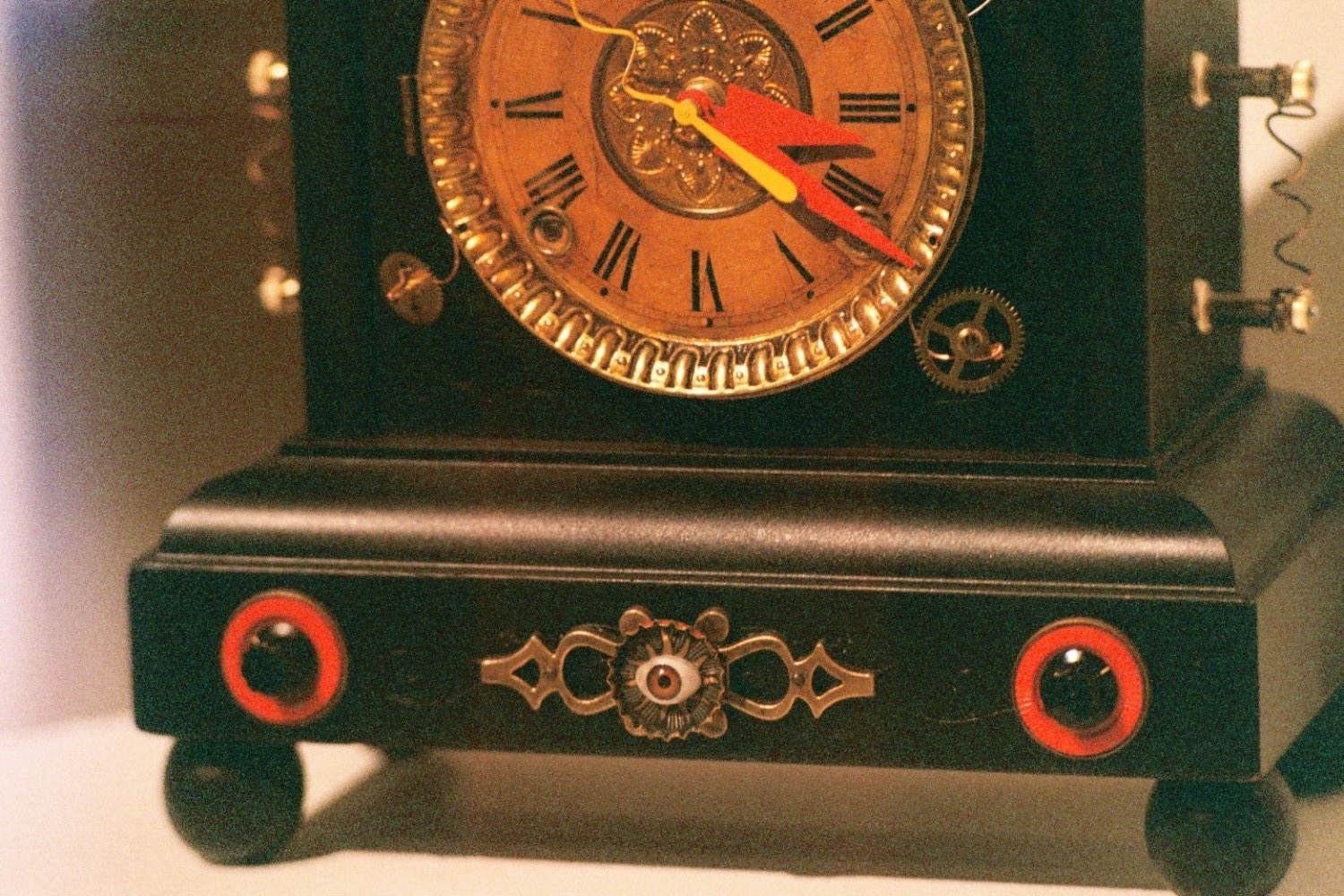This image depicts a vintage clock that may be wind-up or electric in nature. The clock is crafted from dark wood and boasts a face adorned with Roman numerals against an orange-gold background, framed by an ornate golden border. The wooden structure includes a base of the same material, which appears to feature a small drawer, potentially accessible via a central white knob. Flanking the sides of the clock are two red circles, each with a black knob-like feature. The clock stands on four wooden ball feet, one at each corner, providing stability and adding to its antique charm. Both the hour and minute hands are distinctively red, standing out against the decorative face.